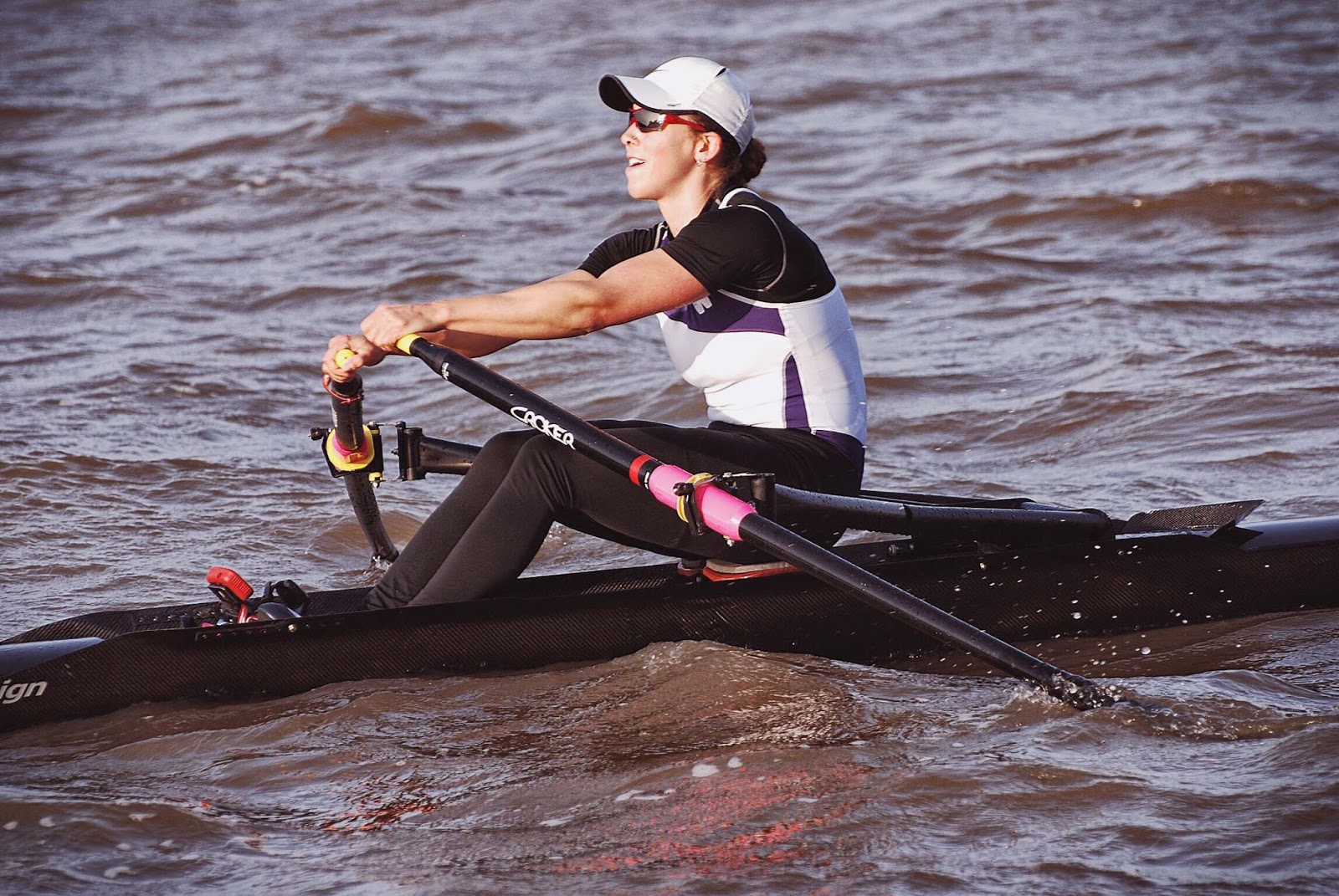In this color photograph, a physically fit woman, who appears to be a professional or semi-professional athlete, is captured in a side profile while rowing a sleek, modern single-passenger watercraft on a body of water with slight waves. The water has a brownish-red hue, potentially reflecting colors from her equipment. She is wearing a white baseball cap with a black underbrim, where her hair is pulled back into a ponytail. She also sports red-framed sunglasses. 

Her athletic attire includes a short-sleeved, form-fitting top with purple and black details, a black undershirt, and black lycra leggings. She wears black shoes or boots. The woman is holding black oars with yellow handles and pink middle connectors, indicating that they might be Croker brand oars. The black watercraft extends beyond the photograph's edges, with a partial inscription showing the letters "IGN." Despite the exertion evident in her tensed arm muscles, she appears to be in good spirits, possibly smiling. This detailed snapshot, taken outdoors in natural daylight, highlights the athlete and her precise rowing form against the textured backdrop of the water.